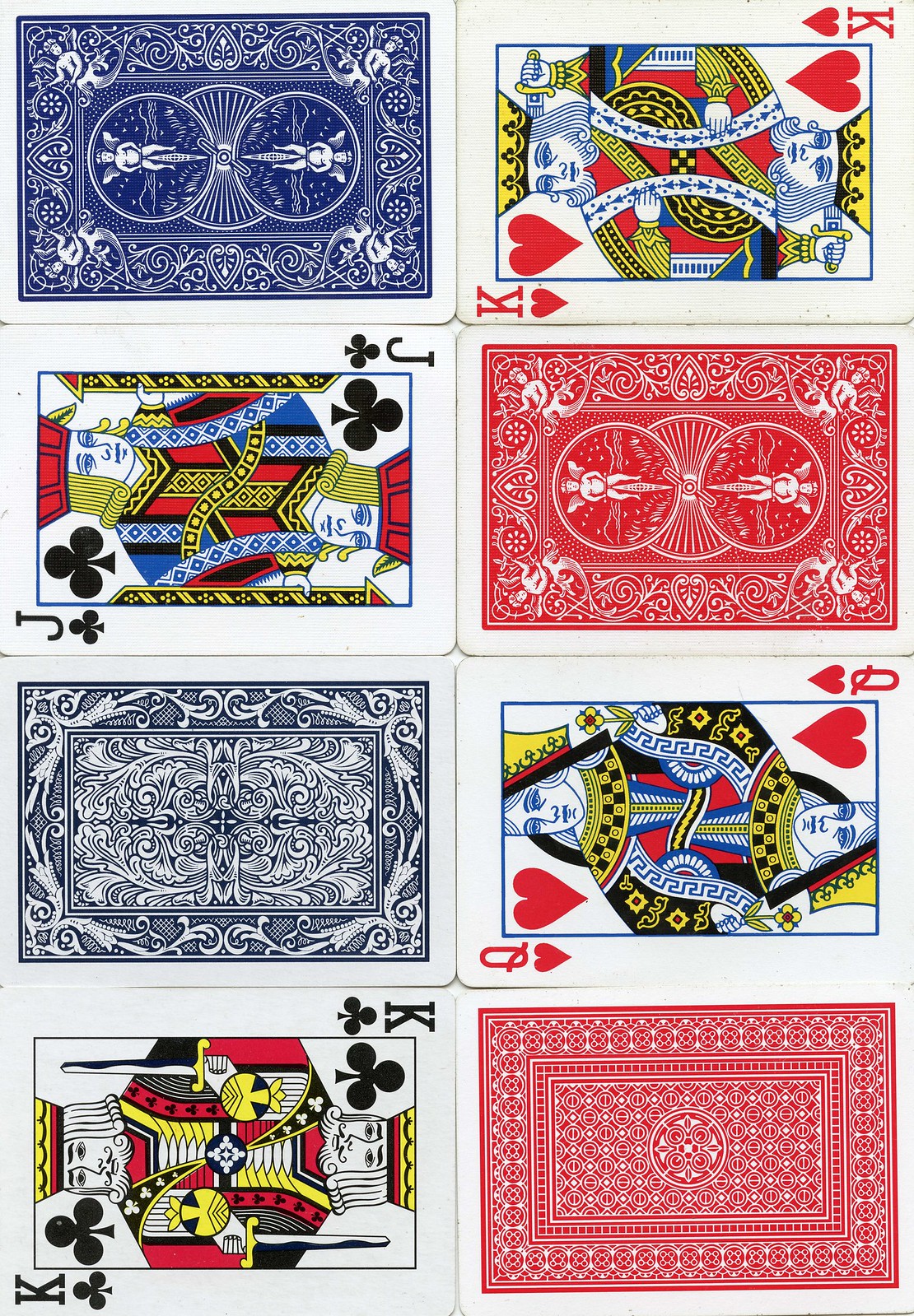In the top left corner of the image, there is a blue card back featuring a detailed design with angel motifs. Angels are positioned symmetrically at the top left, top right, bottom left, and bottom right corners. The center of the card showcases a pattern of three circles, all set against a blue and white striped background. To the right of this blue card, displayed prominently outside the confines of the background design, is a King of Hearts card, with the king illustrated on both the left and right sides of the card.

Towards the middle left, we see a Jack of Clubs card. Adjacent to this is a red card back, mirroring the design of the blue card back in the upper left corner. Just beneath this red card back lies a Queen of Hearts card. Positioned to the left of the Queen of Hearts, there is a card featuring a black background with an intricate square in the middle, adorned with delicate leaf motifs, wave patterns, and other decorative designs.

In the bottom right corner, there is a card with a red background, displaying a central circle and square pattern. Finally, outside the primary arrangement of cards, there is a King of Clubs card set against a white background.